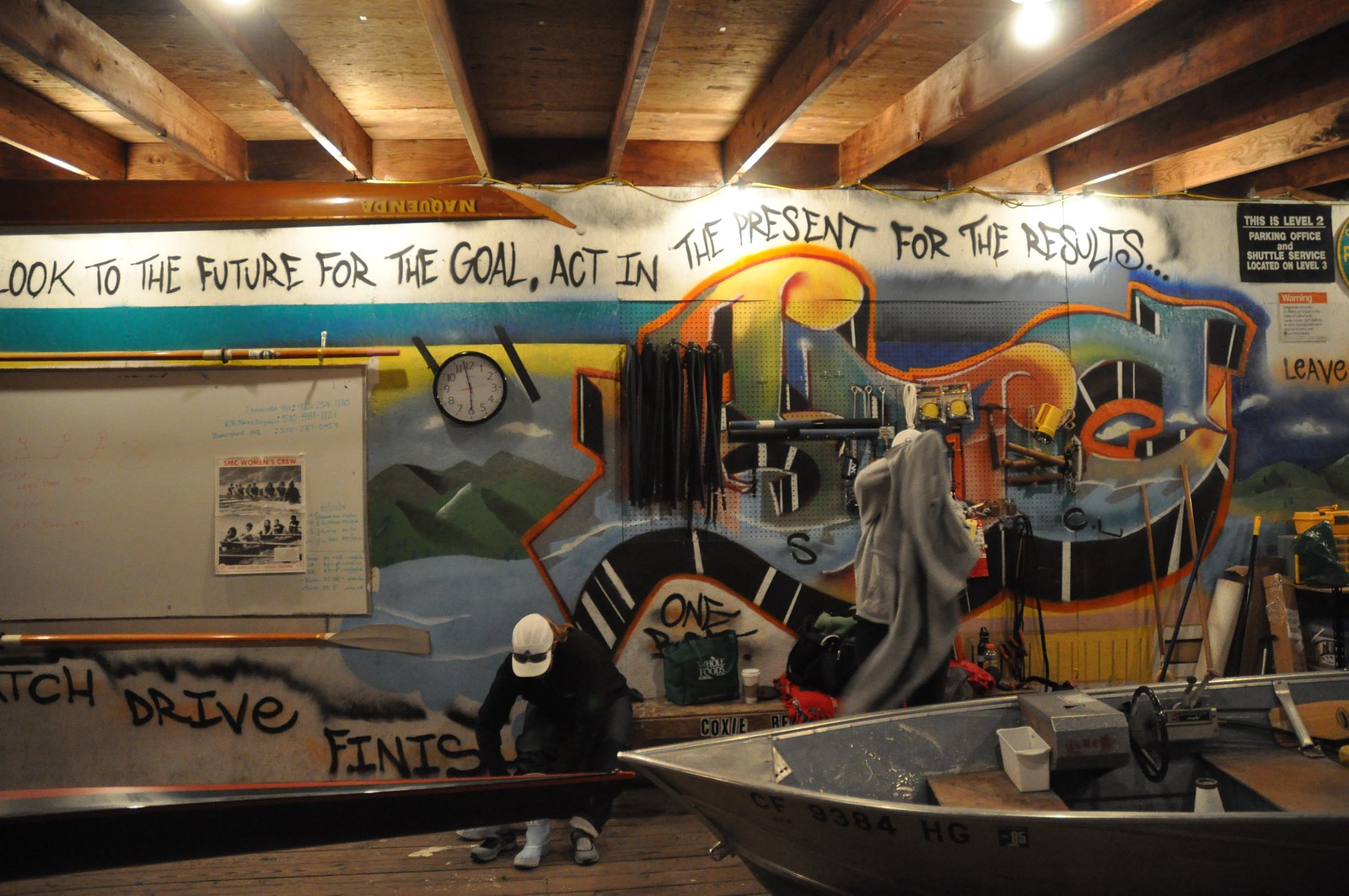The image depicts an unfinished building with a brown wooden ceiling featuring exposed wooden support beams and a few hanging light bulbs. Against the far wall, covered with vibrant street art depicting a river and mountains, there is a pegboard integrated into the mural, holding various tools such as hammers, flashlights, and straps. A whiteboard, framed by boating oars on the top and bottom, hangs on the left side of the wall. The whiteboard has text that reads, "Look to the future for the goal, act in the present for the results." Additionally, there's signage indicating this is "Level Two Parking Office and Shuttle Service on Level Three." The clock on the wall reads 5:57. Positioned in the foreground is a small gray metal boat attached to a trailer, and nearby, a man sits on a bench marked with the letters "C-O-X-L-E." The overall scene includes various elements related to boating and sporting equipment, creating a dynamic and detailed setting.